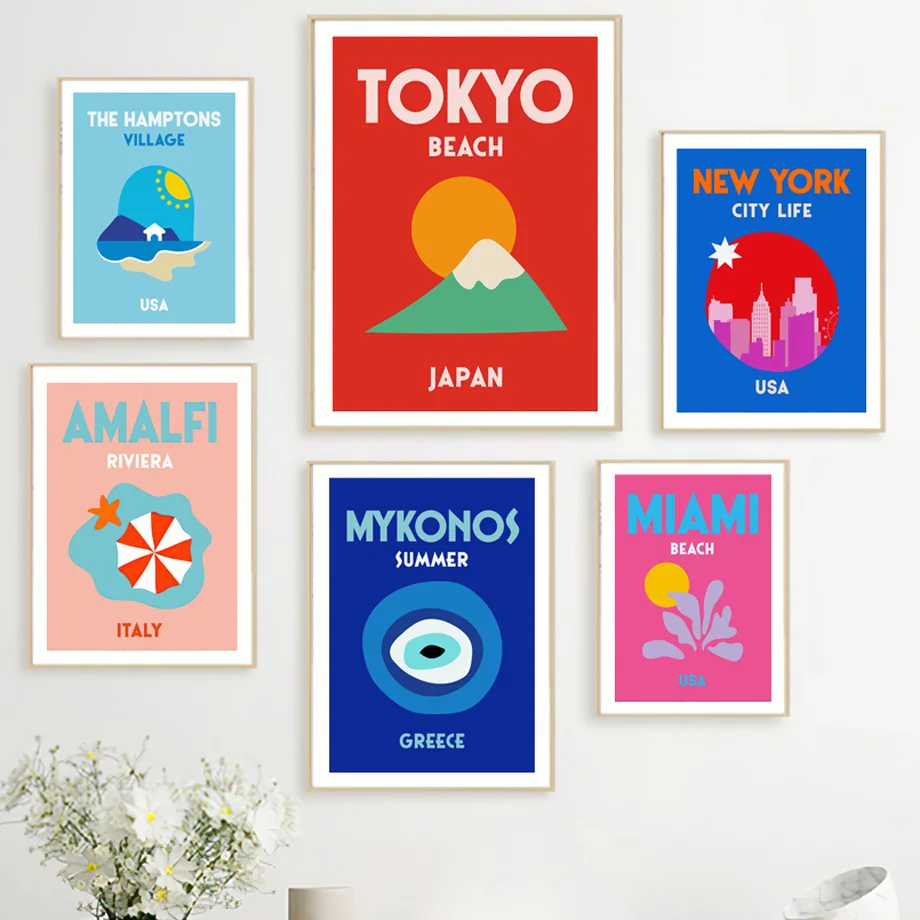An aesthetically pleasing photograph showcases a pristine white wall adorned with six vibrant, colorful pictures. In the lower left-hand corner, a vase with just the tops of daisies peeking out adds a touch of natural beauty to the composition. 

The first image, a rectangular picture titled "Hamptons Village, USA," prominently features a small white house and a sun against a primarily blue background. 

Next, in the middle, hangs a larger rectangular image labeled "Tokyo Beach, Japan." This piece stands out with its predominantly red color palette, showcasing a large orange sun and a green mountaintop capped with snow. 

To the right of this is a smaller rectangular image named "New York City Life, USA." This features skyscrapers in a purple hue set against a blue background, with a striking red circular element in the center. 

In the lower left corner of the picture arrangement, a rectangular image labeled "Amalfi Riviera, Italy" stands against a pink background. The central blue circle contains a red and white umbrella alongside an orange starfish. 

To the right of this, "Mykonos Summer, Greece" is displayed against a dark blue background, featuring concentric circles in light blue, white, aqua, and black for added visual interest. 

Lastly, the image on the far right named "Miami Beach, USA" rests on a pink background. This picture features blue text for "Miami" and includes a small light blue leafy plant against an orange sun. 

Adding to the charm of the image, in the lower right-hand corner, there is a partial view of a white ceramic cup with subtle gray lines, completing the visually delightful scene.